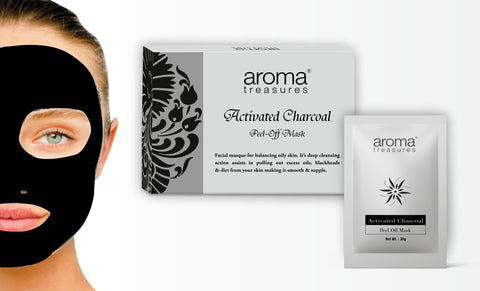This horizontally rectangular advertisement prominently features beauty products against a white background. On the left side, the ad showcases the left side of a fair-skinned woman’s face, partially covered by a black activated charcoal mask. Her blue eye, pink lips, and dark brown hair pulled back are visible. The mask covers her forehead, nose, eye area, and around her mouth, emphasizing the product’s application.

To the right of her face, there are two products displayed. The first is a rectangular box in the middle of the image, featuring the text "Aroma Treasures" in black. Below, it reads "Activated Charcoal Peel-Off Mask," followed by several smaller lines of text, all in black font. Further to the right, there's a single pouch of the same product, also marked with "Aroma Treasures" at the top and additional text underneath. The background transitions from light gray on the right to white on the left, creating a clean, minimalist aesthetic that highlights the product details and the model’s partially masked face.